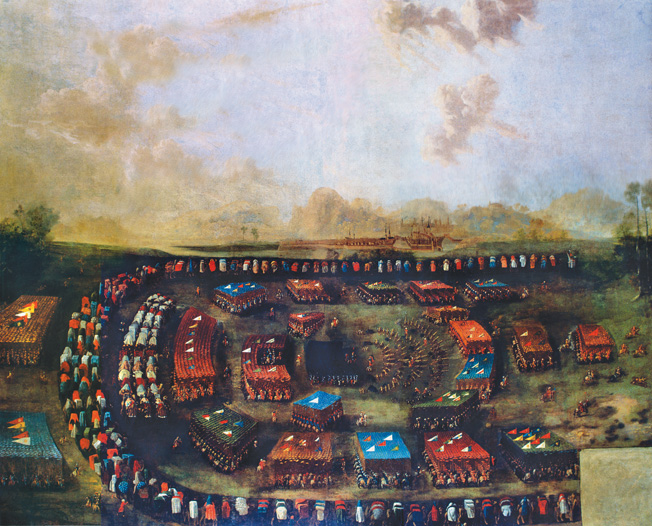The image appears to be an old painting of a large field or grassy plain, bustling with activity. At the center, there are formations of people, possibly soldiers, organized in what could be described as a complex array of patterns. Some formations are in the shape of squares or Cs, with numerous small figures, perhaps marching or standing, creating these shapes. The formations are interspersed with little tents, some larger with blue, flat roofs, surrounded by groups of about four people wide. In the middle, several flags are visible, indicating the significance of these assemblies.

In the background, you can discern a landscape of trees and slight hints of smoke, suggesting campfires or other activities. Near the horizon, there seems to be a large ship with sails, indicating a coastal or riverine setting, or it might be a city with large structures that resemble ships. The sky above is a light blue with brownish clouds, contributing to the overall antique and historical feel of the painting. The scene gives the impression of a military encampment or a large gathering, set against the serene yet intricate backdrop of the countryside.